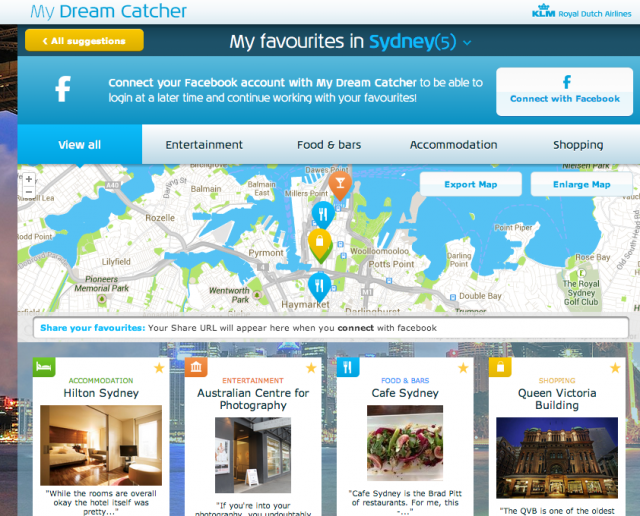Sure, here's a cleaned-up and detailed caption:

---

The image showcases a web page from "My Dream Catcher," an interactive travel planning tool created by KLM Royal Dutch Airlines. The platform allows users to connect their Facebook accounts for seamless login and to save their travel preferences for future access. In this specific example, it highlights "My Favourites" for Sydney, Australia. The page is categorized into sections such as accommodation, entertainment, food and bars, and shopping.

For accommodation, the Hilton in Sydney is featured. The entertainment spotlight is on the Australian Centre for Photography. Under the food and bars category, Café Sydney is recommended, esteemed as "the Brad Pitt of restaurants" by a reviewer. Shopping suggestions include the iconic Queen Victoria Building.

These locations are visually displayed on a map of Sydney, Australia. Users can interact with the map by zooming in, enlarging, or exporting it. Additional navigation options are available at the top, allowing users to refine their search by specific subcategories.